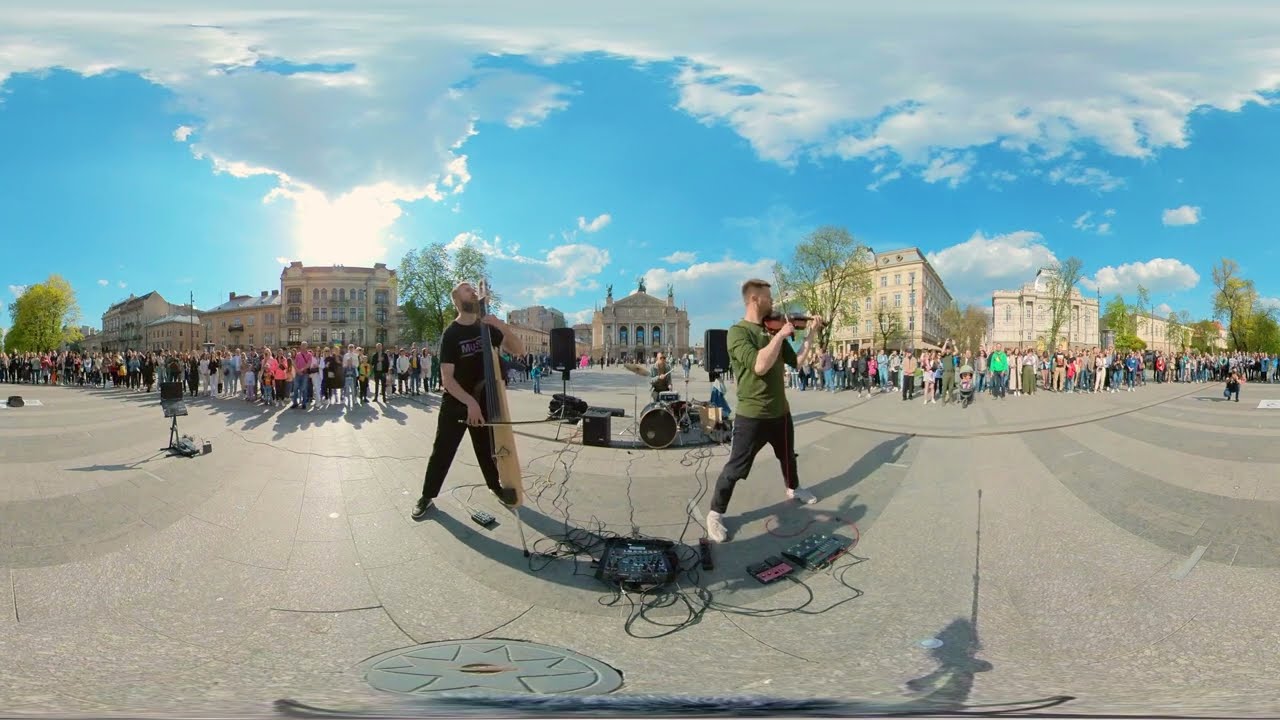In this panoramic fisheye view, we see a vibrant outdoor music scene set against a backdrop of historic buildings under a partly cloudy blue sky. The performance takes place in a courtyard within a European city, surrounded by elegant, low-roofed beige and brownstone buildings, some multi-level with numerous windows. Central to the image are three musicians: on the left, a person dressed in black playing a standing stringed instrument, possibly an electric cello, and in the center-right, another musician in a green shirt, black pants, and white sneakers playing a violin. Behind these two, a drummer with a mohawk and sunglasses is situated in the middle of an array of musical equipment, including black drums, amps, and cords sprawling across the ground. The musicians face the camera, giving the viewer a direct sightline while groups of people stand in the background, enjoying the performance. The scene is lively, capturing a moment where music and urban life intersect harmoniously.